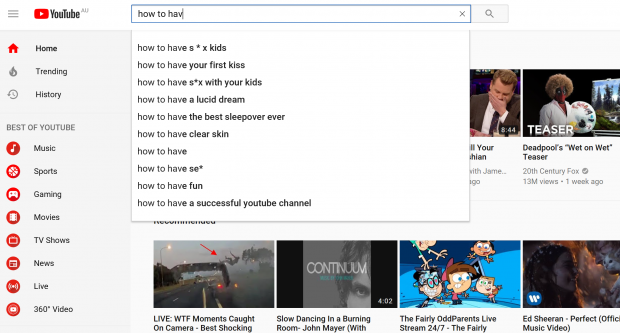This image is a screenshot from YouTube, featuring a distinctive layout typical of the platform. In the upper left corner, we can clearly see the YouTube logo, consisting of a red rectangular icon next to the word "YouTube" written in black text.

Dominating the left side of the screen is the navigation bar, running vertically from top to bottom. The sections listed here include:
- **Home**
- **Trending** (accompanied by an icon of a flame)
- **History**
- **Best of YouTube**
- **Music**
- **Sports**
- **Gaming**
- **Movies**
- **TV Shows**
- **News**
- **Live**
- **360 Videos**

The center top of the screenshot prominently displays a search bar, currently showing the partially entered phrase "How to have." Below the search bar, a dropdown list of autocomplete suggestions is visible. These suggestions include:
- How to have SX kids
- How to have your first kiss
- How to have SX with your kids
- How to have a lucid dream
- How to have the best sleepover ever
- How to have clear skin
- How to have
- How to have SE asterisk
- How to have fun